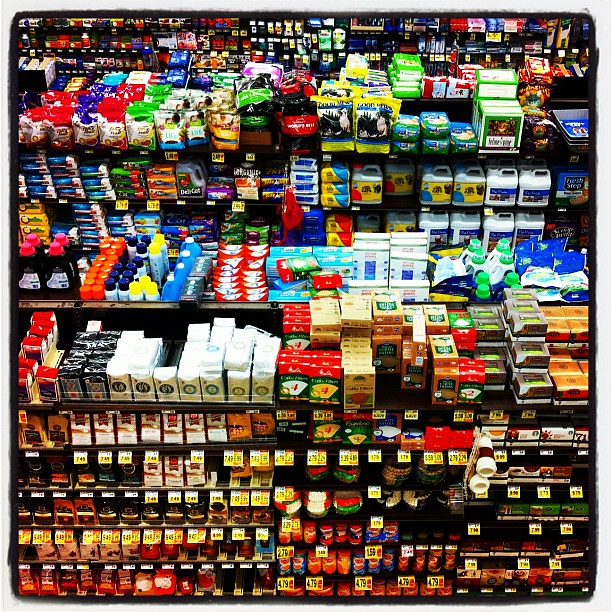The photograph captures the interior of a store featuring multiple aisles stocked with a diverse array of products. Prominently in the image, one aisle displays a variety of packaging in vibrant colors, including blue, red, green, orange, white, and black. On one side of this aisle, there are numerous jugs of cat litter, predominantly of the Tidy Cats brand, which are identifiable by their yellow labels. These jugs come with different lid colors, some blue and some red. Additionally, there are Fresh Step litter packages, easily recognized by the image of an orange cat on the front. The background reveals more aisles filled with brightly colored food packages, enhancing the bustling feel of the store. Price tags on the shelves are noticeable, marked in white and yellow, adding to the detailed organization of the display.